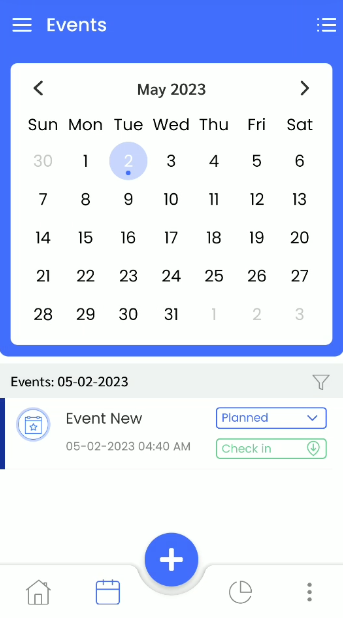This is a screenshot from a mobile phone displaying a partially cut off user interface, seemingly from a calendar application. At the top of the screen, the word "EVENT" is visible. On the left side, there's an icon featuring three horizontal lines, probably indicating a pull-up or slide-in sidebar. Contrastingly, on the right side, another icon with three horizontal lines, each punctuated by a dot on the left side, suggests a different type of sidebar.

Below this, the calendar for May 2023 is outlined in blue. The calendar layout follows the standard format with columns representing Sunday through Saturday, spanning from the 1st to the 31st. Additionally, it includes the 30th from the previous month and the first three days of the subsequent month.

Further down, "EVENTS" is displayed, followed by a specific date of "05-02-2023". Below this, an entry reads "EVENT NEW 05-02-2023 at 4:40 AM" with two buttons labeled "PLANNED" and "CHECK IN" adjacent to this text.

At the bottom center, a blue circular button with a plus sign in its middle is designed for adding a new event. Surrounding this button, there are four icons: a home icon, a calendar icon, a pie chart icon, and an icon with three dots, presumably for additional options or settings.